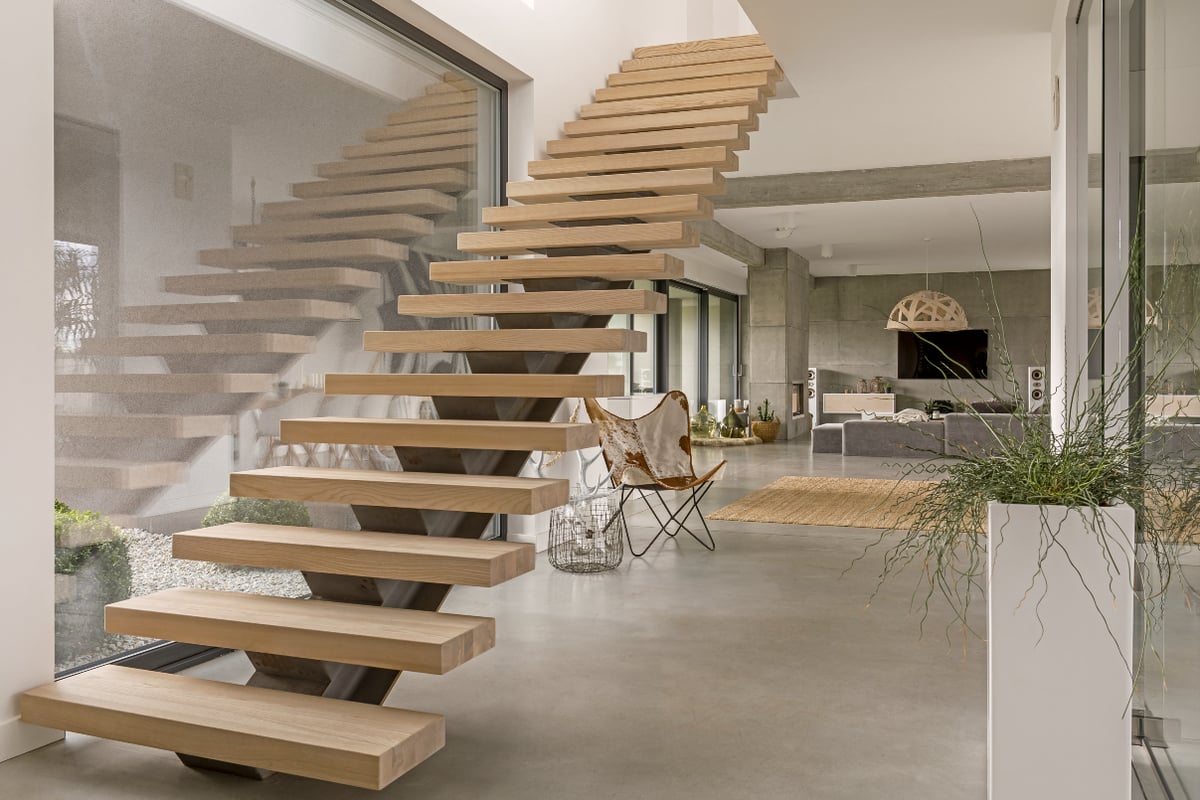In this image, we are looking at the interior of a modern building. On the left-hand side, there is a staircase consisting of 22 rectangular, light brown wooden steps, with a dark gray base supporting it. The room's flooring is a light gray color, complementing the overall neutral tone of the space. To add a touch of nature, there is a vertical rectangular planter with a green plant situated within it. 

Two light gray pillars stand prominently in the room, adding structural and aesthetic value. The décor includes a light brown rug, and a brown and white chair, creating a cozy seating area. At the back, there are several gray sofas, positioned for comfort and style, facing a black rectangular flat-screen TV mounted on the wall. Hanging from the ceiling is a light tan chandelier, adding a touch of elegance and ambient lighting. 

The back wall is painted in a matching gray tone, maintaining the room's cohesive color scheme. On the left-hand side of the room, there is a large, square-shaped mirror, which enhances the space and reflects light. There are also some doors visible towards the far side of the room, suggesting additional rooms or areas within the building. Overall, the room combines modern design elements with functional and stylish furnishings, creating an inviting and sophisticated atmosphere.